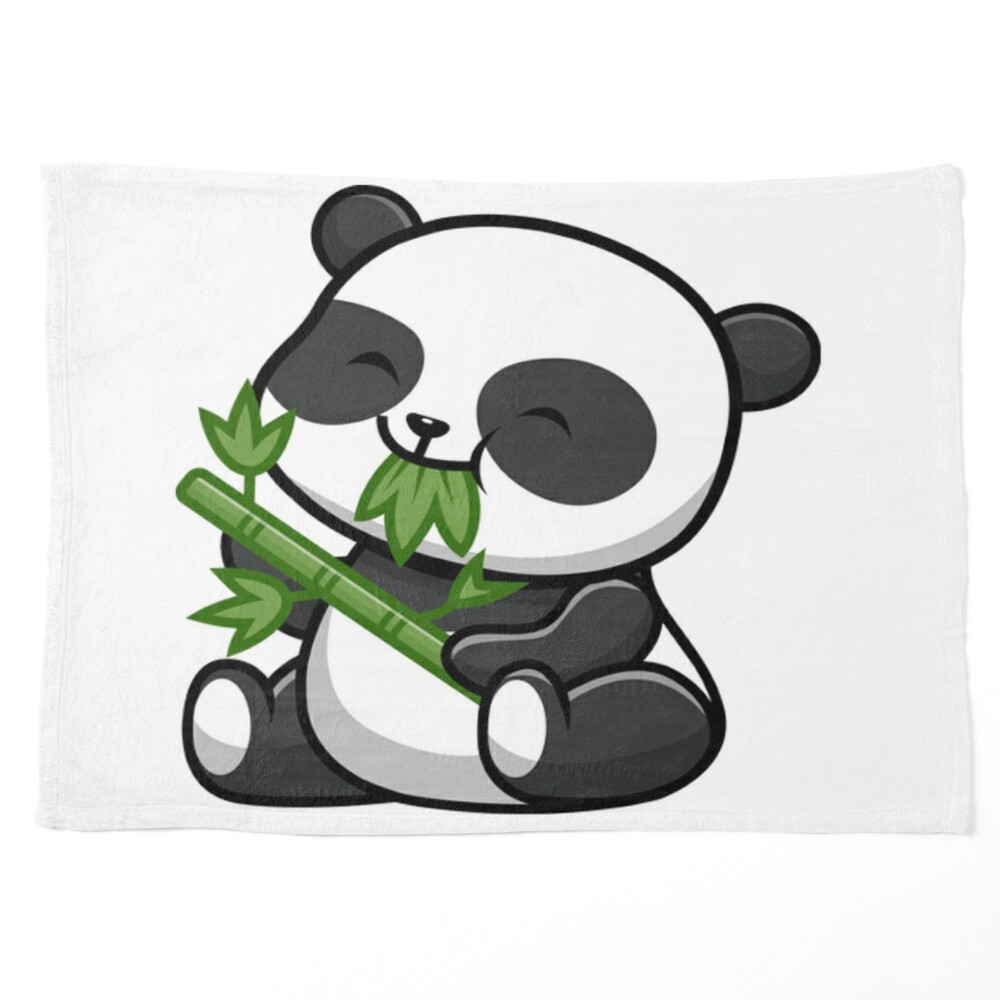This detailed, cartoonish illustration depicts a young, black-and-white panda cub sitting diagonally to the left and delightfully munching on a green bamboo stick. The panda's big smile and eyes curved in joy reveal its happiness, accentuated by a few bamboo leaves sticking out of its mouth. The simple drawing highlights the panda's youthful exuberance as it holds the bamboo with both paws, the stick angled up to the left, with three to five leaves attached. The artwork is printed on a plain, white tea towel, providing a charming contrast between the panda's monochromatic fur and the vibrant green of the bamboo, capturing a moment of sheer panda bliss.